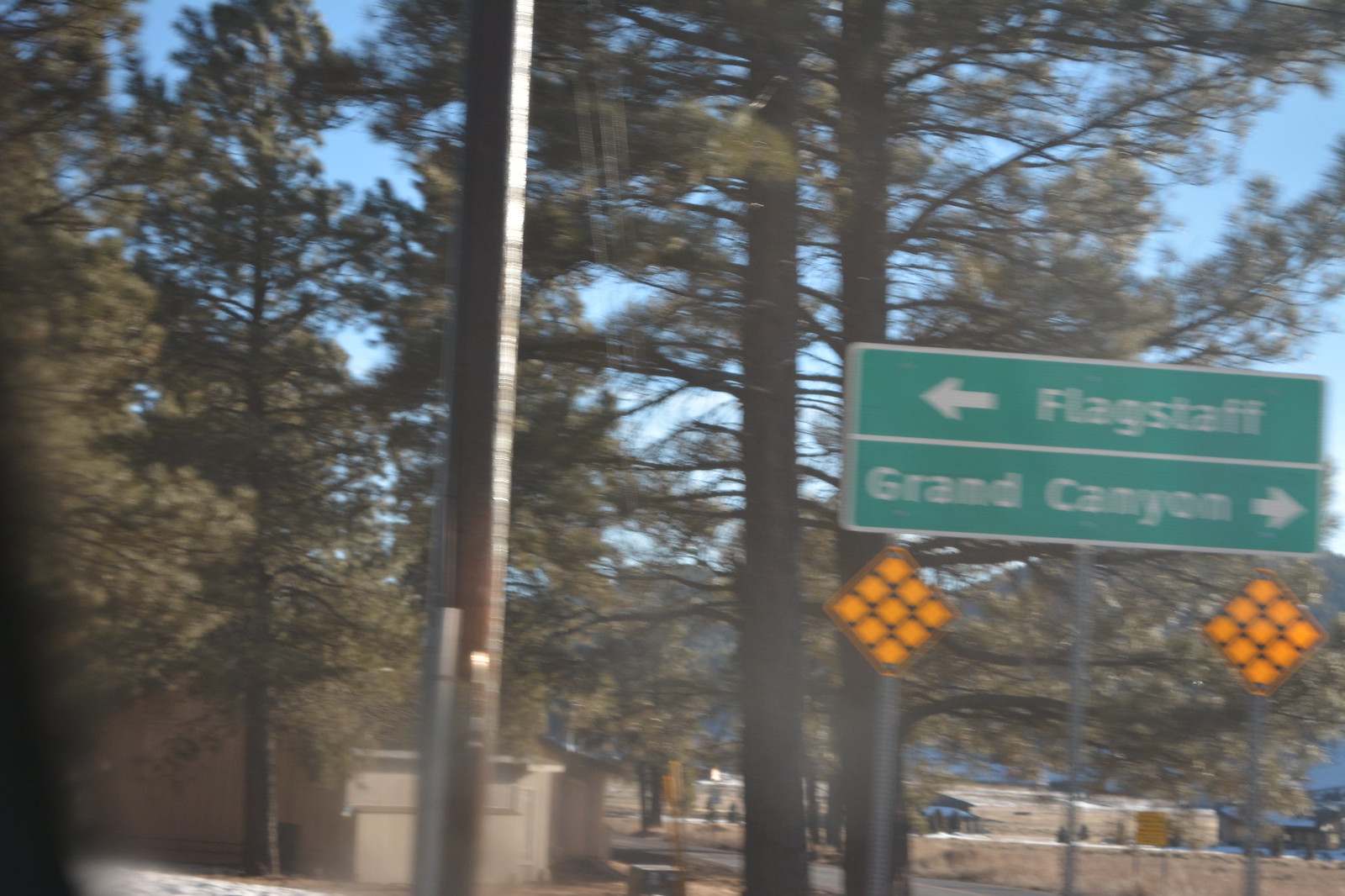The image captures a roadside scene set in an outdoor environment. A prominent green, rectangular sign with a white border stands in the foreground, split vertically by a white line. On the left side of the sign, "Flagstaff" is written in white letters accompanied by an arrow pointing to the left. On the right side, "Grand Canyon" is similarly inscribed with an arrow directing to the right. Below this sign are two diamond-shaped signs with a yellow background and black, honeycomb-like lines. The background features large pine trees reaching towards a clear blue sky. A power pole is positioned slightly to the left of the sign. In the lower right corner, a brown building is partially visible. Additionally, another building with a lighter gray-brown coloration is noticeable behind the power pole, further reinforcing the setting's rustic charm.